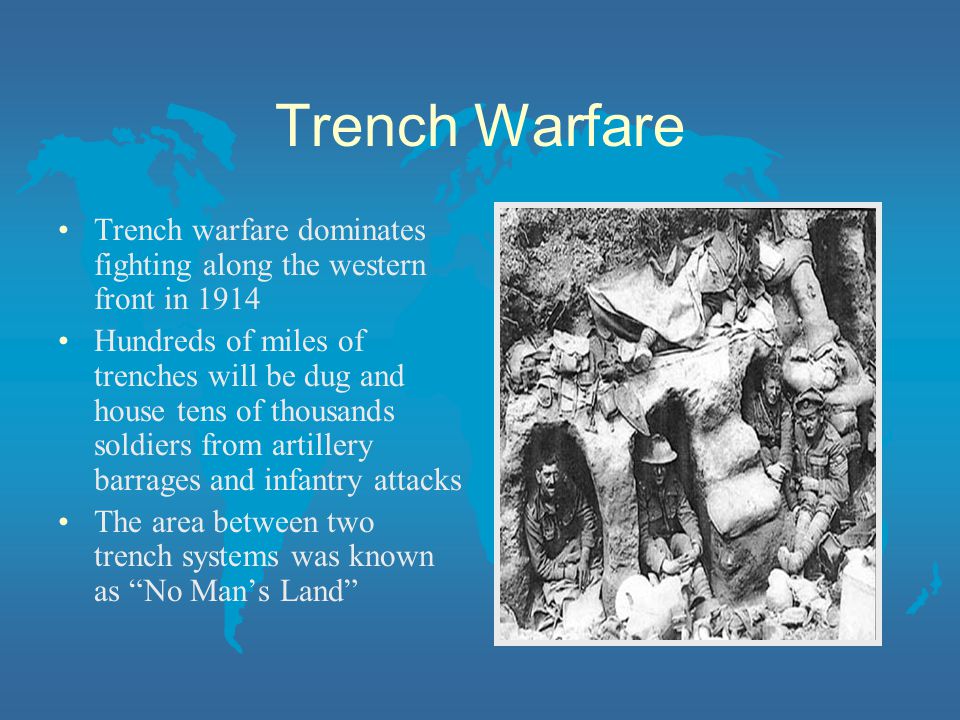The image appears to be a still from a PowerPoint presentation with a blue background featuring a lighter blue map of the world. At the top, white letters prominently display the title "Trench Warfare." On the left side of the slide, bullet points describe key aspects of trench warfare: it dominated the fighting along the Western Front in 1914, with hundreds of miles of trenches dug that housed tens of thousands of soldiers, providing shelter from artillery barrages and infantry attacks. The area between two trench systems was known as "no man's land." To the right of these bullet points, there is an old black-and-white photograph showing life in the trenches. The photo features several soldiers, likely four or five, positioned within the trenches, which appear well-concealed. The entire slide seems to be part of a detailed educational presentation on trench warfare during World War I.